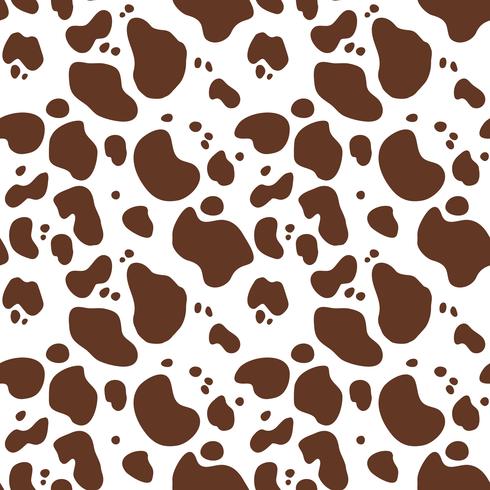The image is a square graphic featuring a distinctive pattern of dark brown spots on a stark white background. These spots are highly irregular in shape, resembling natural forms such as kidney beans, wooden art palettes, or even figure-eights that appear slightly stretched and tilted. The largest spots are about 1/8 to 1/10 the length of the image's side, with much smaller ones interspersed throughout, none larger than an eighth the size of the largest spots. None of the brown spots are perfectly circular; instead, they have varied, quirky edges, reminiscent of cow spots. The design lacks any additional elements or outlines, focusing solely on this scattered, naturalistic pattern which could be suitable for background graphics or other design work.